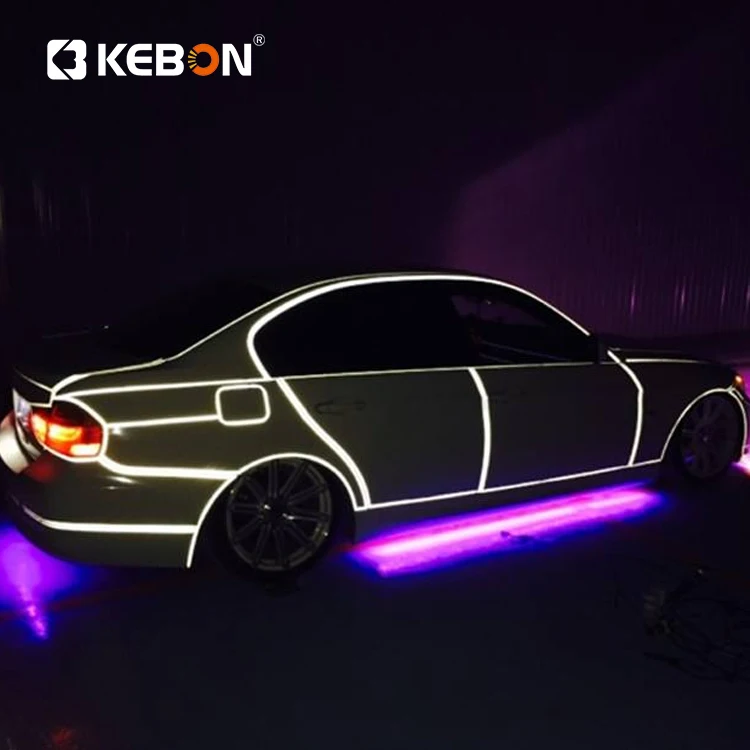This image features a futuristic-looking sedan captured from the perspective of the passenger side rear wheel, angled towards the front end of the car. The sleek black vehicle is set against a dark blue backdrop, heightening its modern aesthetic. The car's outline is accentuated with white, reflective highlights that trace around the doors, windows, roofline, gas tank, rear lights, and bumper, as well as the hood and wheel wells. These white lines give the vehicle a glowing effect, reminiscent of black light illumination. Beneath the sedan, pink and purple LED lights are mounted below the passenger doors and rear bumper, casting a vivid glow on the ground underneath. The backlight of the car also shines with yellow and red hues. The brand "Kebon," with a distinct red 'O,' is prominently displayed in the upper left corner, indicating this image might serve as an advertisement. The overall scene, with its dark surroundings and strategic lighting, emphasizes the car's advanced and stylish design.